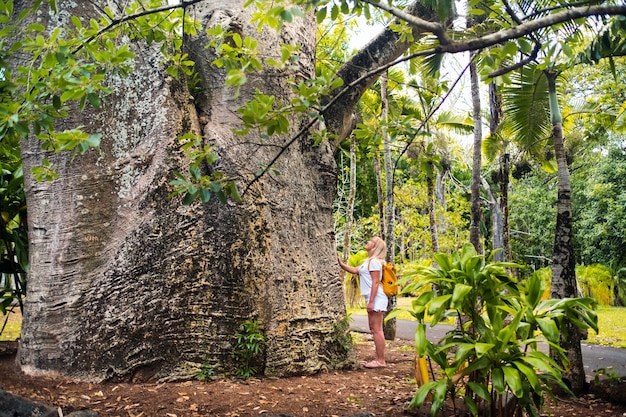In the vibrant color photograph, a majestic, ancient tree with a trunk as wide as a car stands prominently in the center, its sprawling branches adorned with lush green leaves. To the right of this colossal tree, a young blonde woman dressed in a white t-shirt and short white shorts, with a yellow backpack slung over her shoulders, touches the tree trunk with her right hand. She gazes upward, her expression filled with wonder, emphasizing the immense scale of the tree. She appears to be wearing sandals. Scattered around are various other trees and green plants, but none as imposing as the central tree. The ground beneath her feet is bare dirt, and a paved walkway stretches behind her, leading to a tree-lined horizon. The photograph captures a sunny day, with no other people visible, allowing the viewer to fully appreciate the serene, natural beauty of the scene.